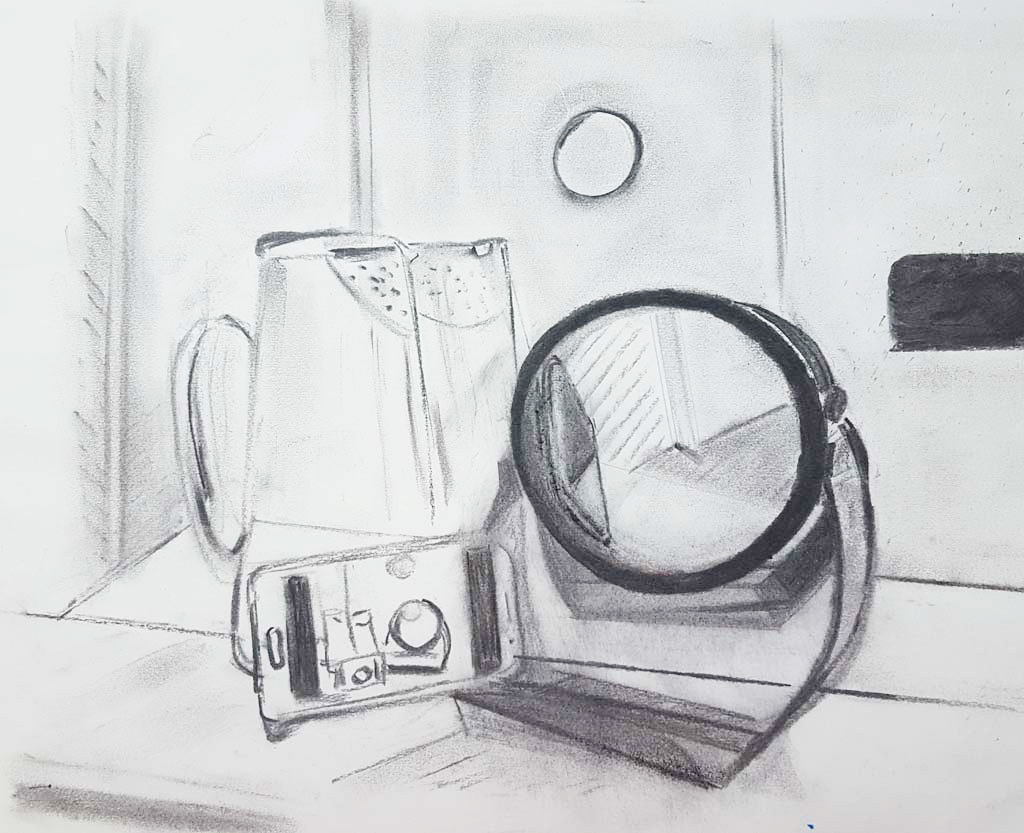This image features a detailed charcoal drawing on a plain white sketch pad. Centered on the page is a round vanity mirror with a strap, reflecting an unseen part of the room. To the center right is a black rectangular object, partially cropped. In front of the mirror, there is an arrangement of items on a platform suggested by three lines running from the lower left to the lower right. These items include a detailed purse with a circular handle, a glass pitcher filled with water and citrus slices, and a smartphone that intriguingly contains a miniature image of the scene. Behind these objects, a wall with a circular porthole-style window adds depth to the composition. The delicate interplay of objects and reflections creates a complex and engaging still life.